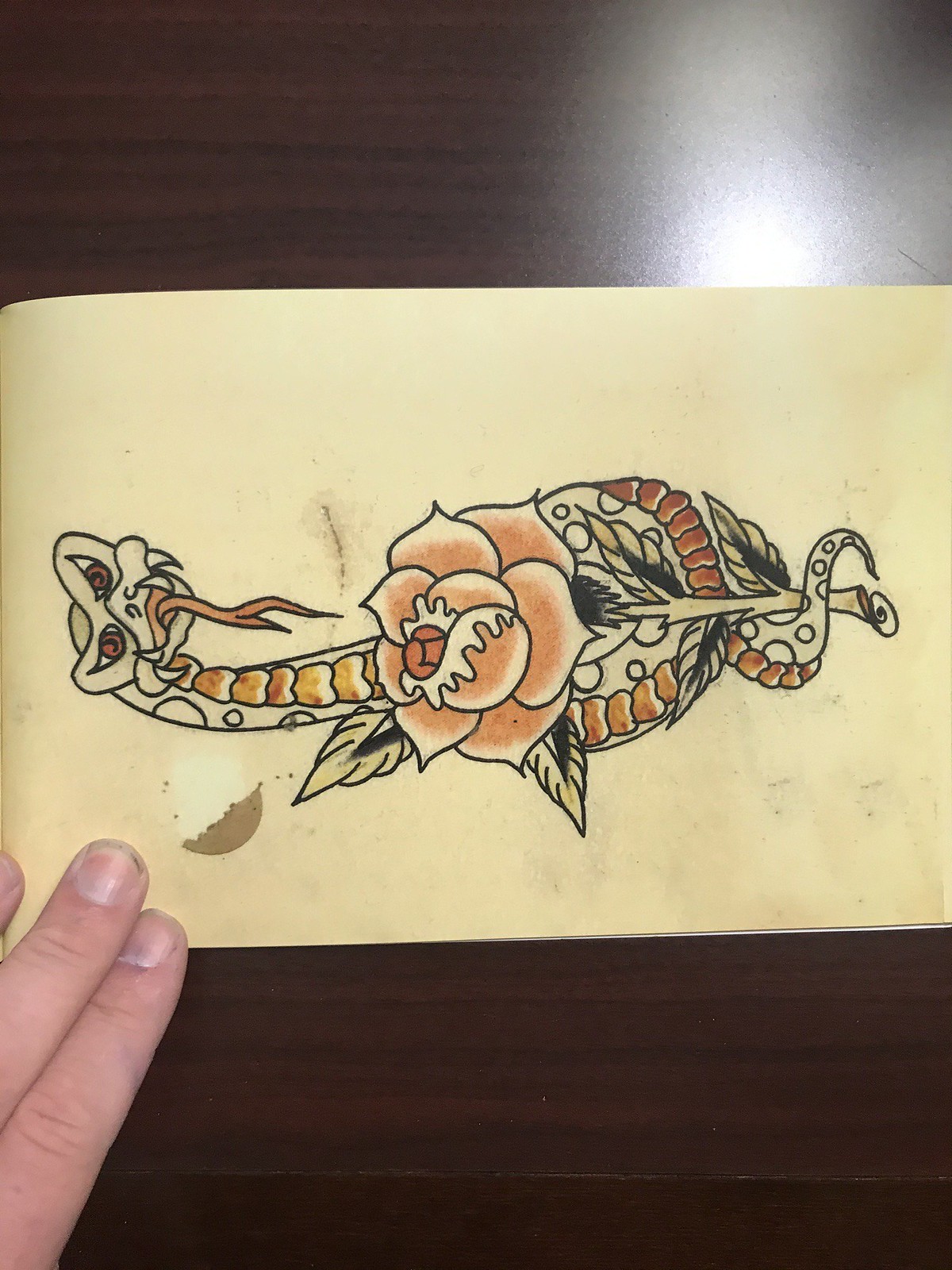This enchanting illustration features a whimsical baby dragon with its head curiously turned over its shoulder, gazing directly at the viewer. The dragon is rendered in a blend of pink, brown, black, and white hues, creating a strikingly decorative appearance. Its body and tail, which extends gracefully behind it, are adorned with distinct round circular patches that contribute to its fantastical charm. The artwork is held steady by three human fingers visible at the bottom, securing the piece of paper in place. Notably, the dragon's legs are absent from the drawing, and an unusual, unidentified element emerges from one side, adding an intriguing and mysterious quality to the scene.